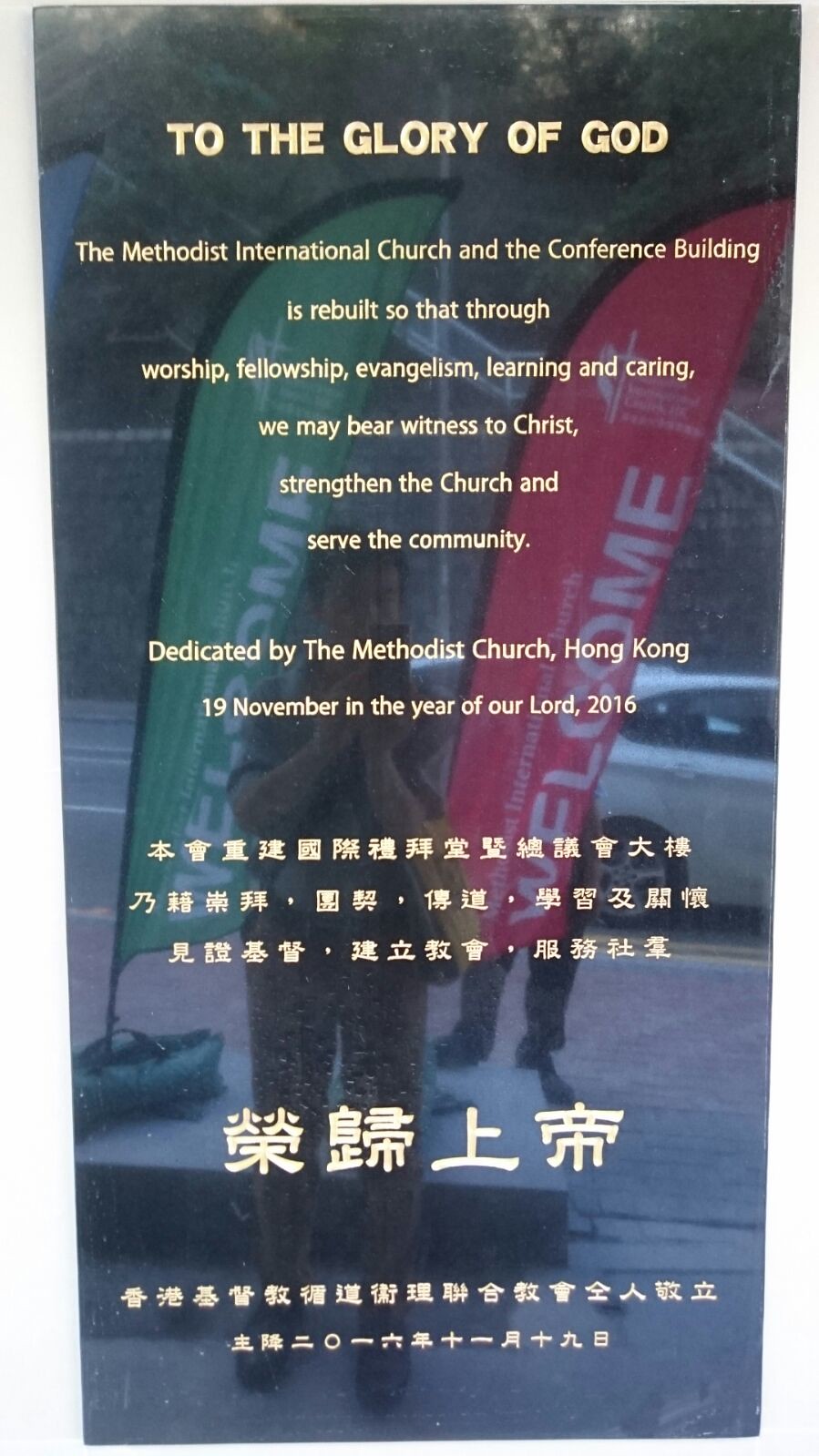The image captures a reflective moment of a person standing outside, seemingly taking a selfie with their phone held in both hands. The photo, slightly blurry and lacking vibrant colors, shows their reflection against a dark plaque with yellow writing. The plaque reads: "To the glory of God, the Methodist International Church and Conference Building is rebuilt so that through worship, fellowship, evangelism, learning, and caring, we may bear witness to Christ, strengthen the church, and serve the community. Dedicated by the Methodist Church, Hong Kong, 19 November in the year of our Lord 2016." Below the English text, there is additional writing in Chinese characters. Behind the person, there are green and red flags that say "welcome," set against a backdrop that includes a white car parked on a brick sidewalk, trees in the distance, and a brick wall.